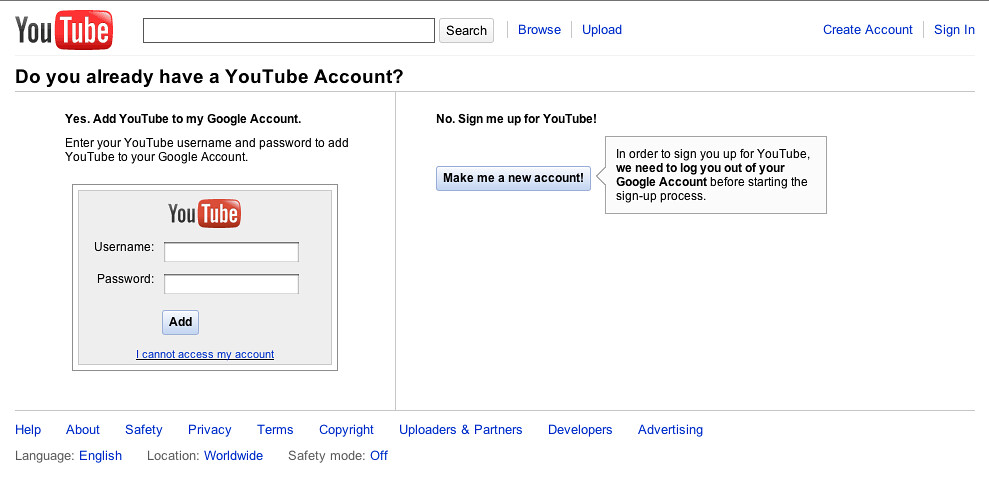The screenshot captures a page on YouTube's website, emphasizing various user interaction elements and account management options. In the upper right corner, the YouTube logo is prominently displayed, featuring "YOU" in black letters followed by a red square with "Tube" written in white, reminiscent of a speech bubble. Adjacent to the logo is a long, empty rectangular search field, and to its right, a button labeled "Search." Further right, there are blue links with the texts "Browse" and "Upload." Continuing to the extreme right, there are additional blue links for "Create Account" and "Sign In."

Below the YouTube logo on the left side, the page prompts users with the question, "Do you already have a YouTube account?" Followed by the statement, "Yes, I add YouTube to my Google account. Enter your YouTube username and password to add YouTube to your Google account." Below this message is a grey box containing the YouTube symbol and fields for entering a username and password, accompanied by an "Add" button. At the bottom of this section, there is a link stating "I cannot access my account."

To the right of this section is another area, separated by a grey bar. It begins with the option "No, sign me up for YouTube," and below this is a blue button labeled "Make me a new account." Next to this button is a rectangle with black text, explaining, "In order to sign up for YouTube, we need to log you out of your Google account before starting the sign-up process."

At the bottom of the page, blue text links provide additional resources with labels: "Help," "About," "Safety," "Privacy," "Terms," "Copyright," "Outperson," "Partners," "Developers," "Advertising." Just above these links, there is information regarding language, location, and safety settings: "Language" displayed in grey followed by "English" in blue; "Location" in grey followed by "Worldwide" in blue; and "Safety Mode" in grey followed by "Off" in blue.

The overall design is user-centric, aiming to guide users through the process of managing and creating a YouTube account with clear instructions and accessible links.